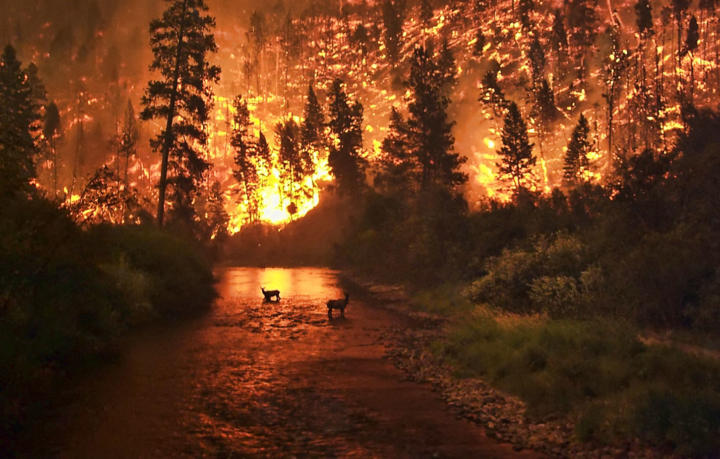The photograph captures a nocturnal scene that seems to be set amidst a forest in the midst of a raging fire. In the foreground, two deer are standing in a shallow river, the water barely reaching up to their feet, as they appear to be attempting to escape the blaze. Surrounding the river, greenery flourishes on both banks, with trees and shrubbery that have not yet succumbed to the fire. In the background, an intense forest fire engulfs the trees, spreading across what looks like a steep hillside or mountain. The flames are vibrant and orange, creating a stark contrast against the dark night sky. Embers and bright flames can be seen behind the trees, contributing to the atmosphere of urgency and danger. The haunting image, dominated by the fire's bright glow, evokes a sense of terror and desperation as the deer gaze toward the camera, seemingly confused and frightened by the encroaching inferno.